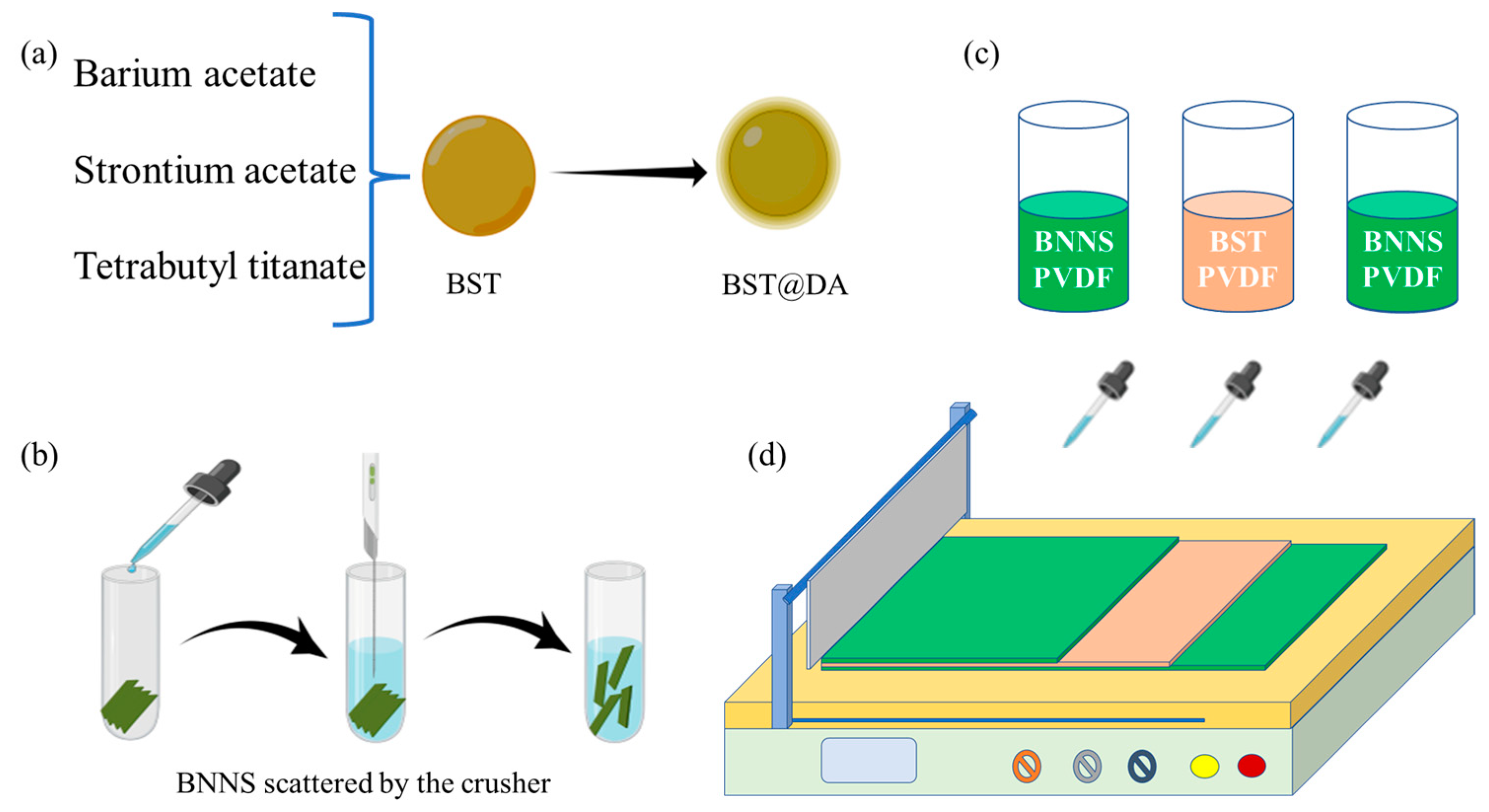The image depicts a detailed scientific diagram segmented into four labeled parts: A, B, C, and D. 

In the top left (A), it specifies the compounds barium acetate, strontium acetate, and tetrabutyl titanate, all linked by a blue bracket to an orange circle labeled “BST.” This orange circle is further connected by a black arrow to a lighter orange circle labeled “BST at DA.”

In the bottom left (B), three test tubes are illustrated. The first test tube shows a water dropper adding water to some green material inside, labeled as BNNS. An arrow points to the second test tube, where the green particles are dispersed in the water. The final test tube shows the particles completely broken down and scattered, labeled as "BNNS, scattered by the crusher."

In the top right (C), three cylinders are filled halfway with different colored substances. The first and third cylinders, filled with green material, are labeled "BNNS, PVDF." The middle cylinder contains a peach-colored substance, labeled "BST, PVDF." 

In the bottom right (D), a machine is depicted with blue, green, and pink materials positioned above it, with dropperfuls of water placed over them, suggesting a process involving these materials with the machine, possibly involving measurement or treatment.

This composite representation outlines the preparation and characterization processes of various compounds and materials in a scientific experiment.